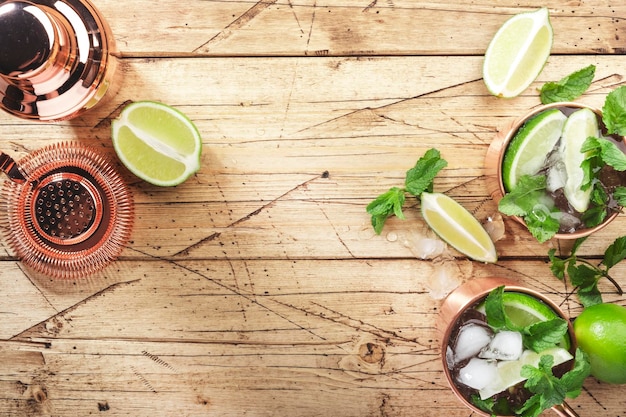The photo depicts a well-worn bar counter or wooden surface, possibly serving as a cutting board, with numerous knife marks and scratches. Scattered across the table are multiple lime slices, some face up and some face down, alongside sprigs of fresh mint leaves and ice. Prominently featured are copper mugs and a copper-colored cocktail shaker with its strainer lid, placed towards the top left. These copper vessels, traditionally used for serving Moscow Mules, each contain a beverage garnished with lime slices and mint. Additionally, there are small pink saucers with accompanying bowls that contain tiny round brown items, possibly resembling caviar, with a half lime slice positioned nearby. The overall setting suggests a detailed preparation area for cocktails requiring lime and mint, highlighting an atmosphere of casual yet meticulous mixology.